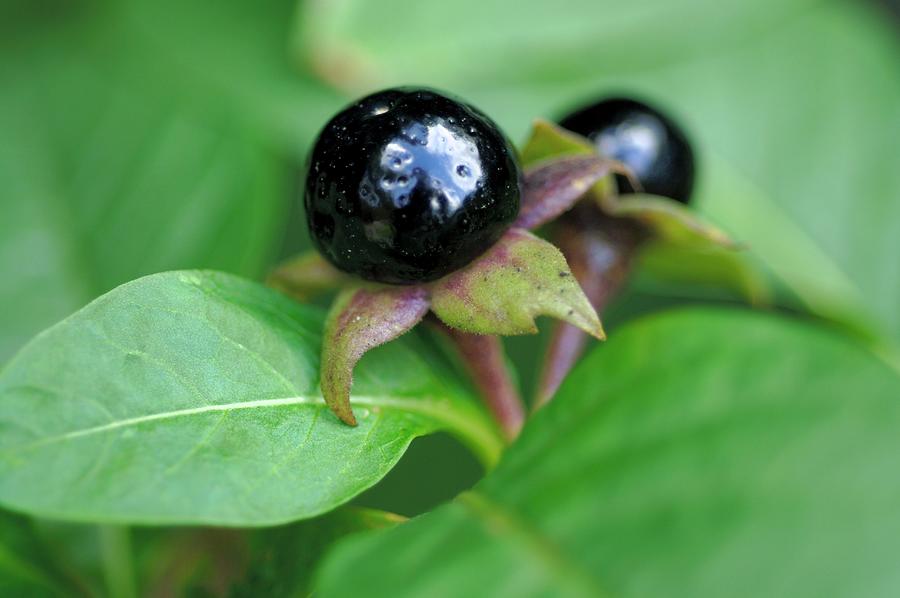This image captures an ultra close-up of a berry plant with exquisite details. At the focal center is a dark, glossy berry, possibly a blueberry, perched on vibrant green leaves. The smooth surface of the berry is adorned with tiny pockmarks and white stains, suggesting it may not be fully mature. Two prominent leaves cradle the berry, with several more blurred in the background, enveloping the scene in greenery. The berry appears to be emerging from a light brown stem with white trim, positioned above the remnants of a small flower. In the backdrop, another berry comes into view, though it is out of focus. The composition emphasizes the lush, bright green foliage and the intricate textures of the fruit, encapsulating the essence of burgeoning nature.